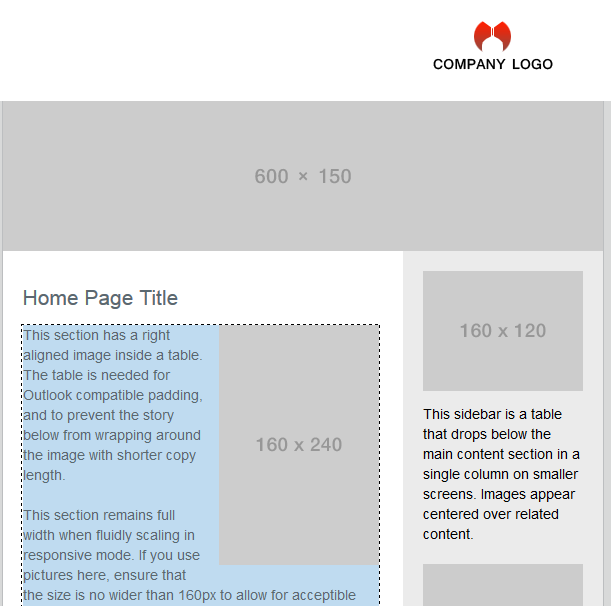This image is a detailed screenshot of a website template designed for structural guidance. The very top features a white border, and in the upper right-hand corner, "COMPANY LOGO" is written in medium gray, capital letters, indicating where the actual company logo should be placed. Accompanying this text is a small red circular image with cutouts at the top and bottom, resembling a white hourglass within the circle.

Directly beneath this header is a light lavender, or perhaps light gray, rectangle that spans the full width of the template, labeled with the dimensions "600 x 150". This area seems designated for a particular banner or image size.

Below this, the main body of the template has a white background. On the left side, there is a heading "Homepage Title" and a square that combines a sky-blue background with a smaller insert in the upper right-hand corner in the same lavender-gray hue as above. This section carries a descriptive label, "This section has a right-aligned image inside of table," providing details on its intended use.

On the right side of the main body, a square area is marked with dimensions "600 x 120". Below this, there's a description: "This sidebar is a table that drops below the main content section in a single column on a smaller screen," which explains that the sidebar will adjust responsively. Additionally, it notes, "Images appear centered over related content," describing how images will be displayed within the content.